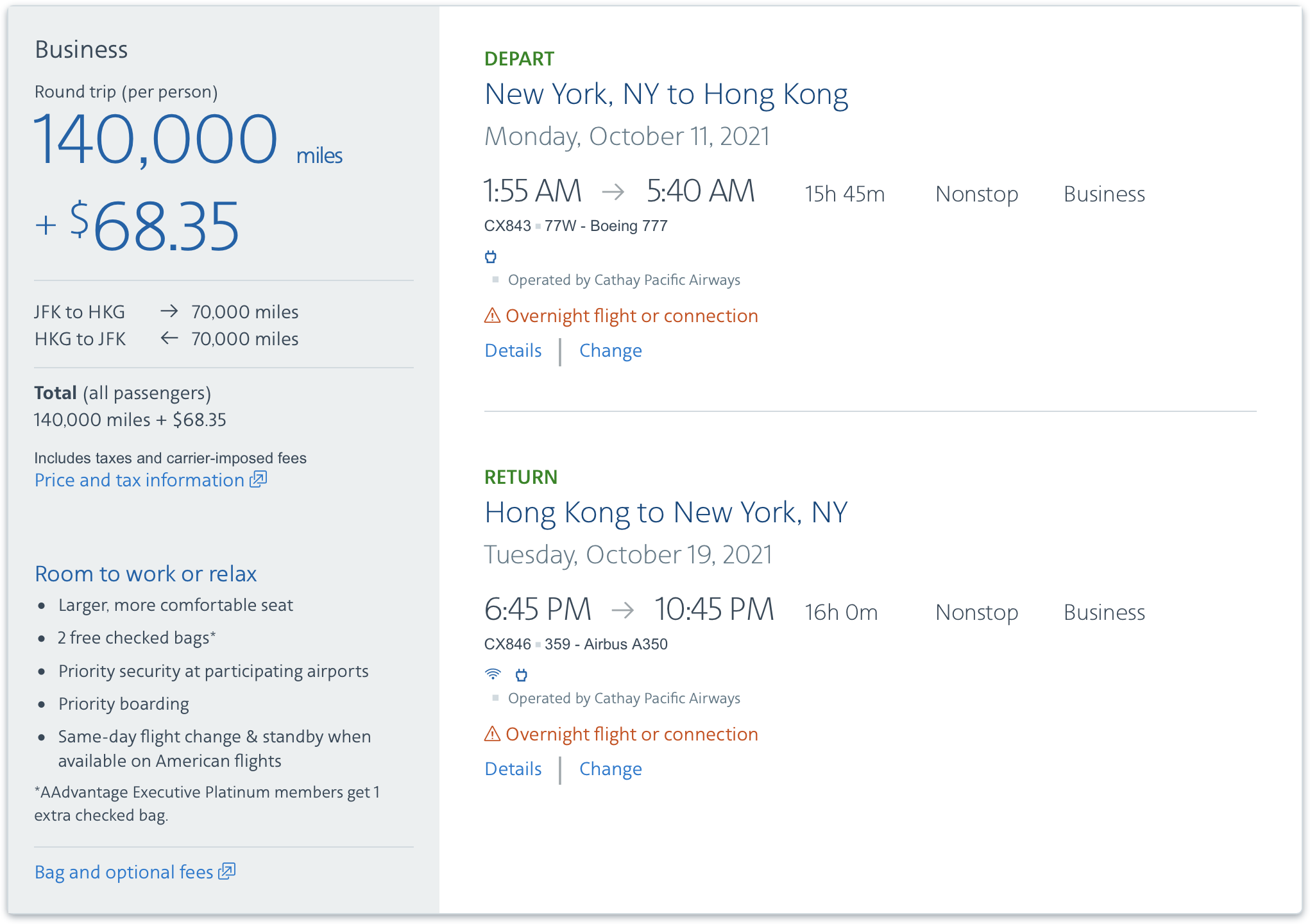**Detailed Descriptive Caption:**

The image appears to be a screenshot of a computer display showing a flight booking summary. On the far left, within a gray-bordered section labeled "Business," it is detailed that the round trip cost is 140,000 miles plus $68.35 per person. The itinerary lists a departure from JFK (John F. Kennedy International Airport) to HKG (Hong Kong International Airport) covering a distance of 70 miles each way. The total mileage for all passengers is stated to be 140,000 miles, in addition to the $68.35 fee.

Beneath this, there are various business class amenities listed, including: 
- "Room to Work or Relax" 
- "Larger, More Comfortable Seat"
- "Two Free Checked Bags"
- "Priority Security at Participating Airports"
- "Priority Boarding"
- "Same Day Flight Change and Standby When Available on American Flights."

At the very bottom left, there is a link labeled "Bag and Optional Fees" highlighted in blue.

The right side of the screen contrasts in white, presenting the detailed flight schedule. The "Depart" section is highlighted in green, showing a flight from New York to Hong Kong on Monday, October 11th, 2021, departing at 1:55 a.m. and arriving at 5:40 a.m. Alongside this, specific time and flight information are provided.

For the return trip, it lists a flight from Hong Kong to New York on Tuesday, October 19th, 2021, with a departure time of 6:45 p.m. and an arrival time of 10:45 p.m. Similar to the departure details, the return section also includes relevant time and flight information below the date and time.